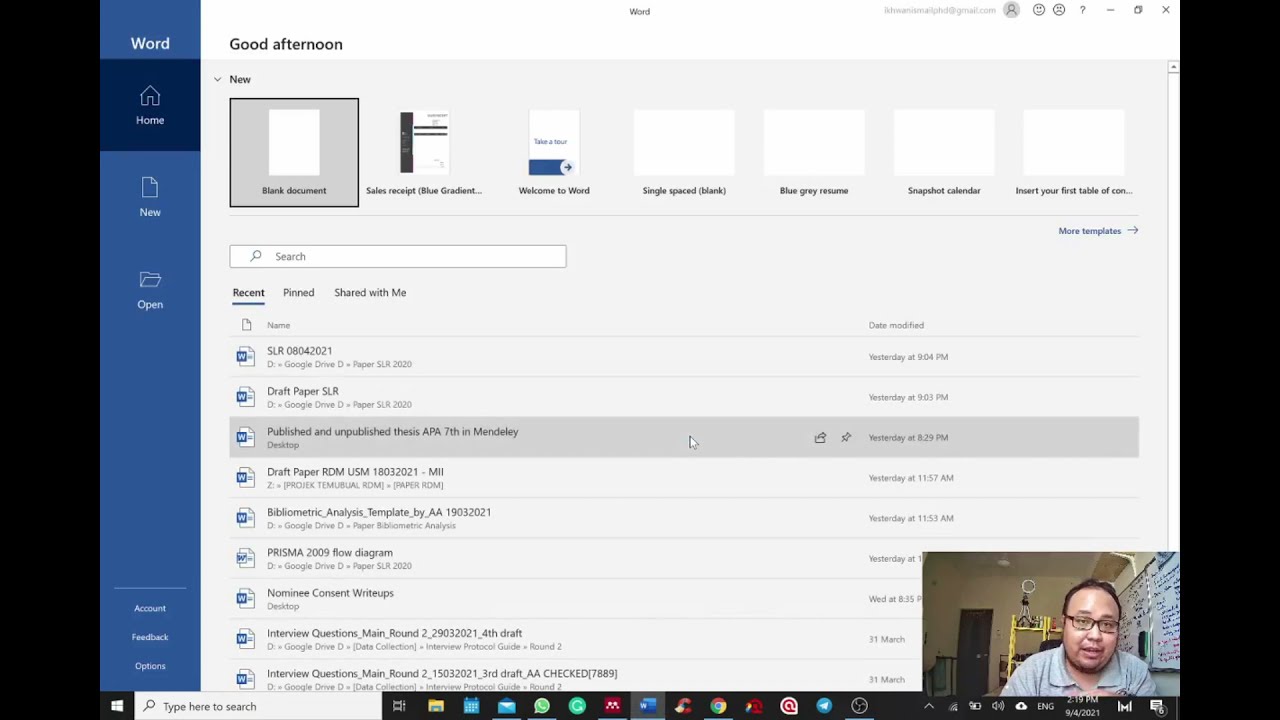This image captures a detailed scene focused on a Microsoft Word tutorial, likely being streamed online. The image features a user interface with distinct black strips framing both the left and right sides. Adjacent to these, on the left, runs a blue strip with "Word" written in white letters at the top. Beneath this, a darker blue strip spans horizontally, displaying icons such as a home, house, and a folder, all in white on a blue background, labeled "Home," "New," and "Open," respectively. Below are various options like "blank document," "published and unpublished thesis," and "APA 7th in Mendeley."

In the bottom right corner, a small video window reveals an Asian man, slightly overweight with thin black hair, wearing black-framed glasses and a gray collared shirt. He appears to be guiding viewers through the Word interface, suggesting he might be an educator or trainer. The taskbar at the bottom confirms the Windows operating system, hinting at an HP device. Notably, on the wall behind him, there's a large whiteboard filled with writing, reinforcing the tutorial atmosphere. His mouse is seen highlighting a recent document, indicating active engagement with the Word application.